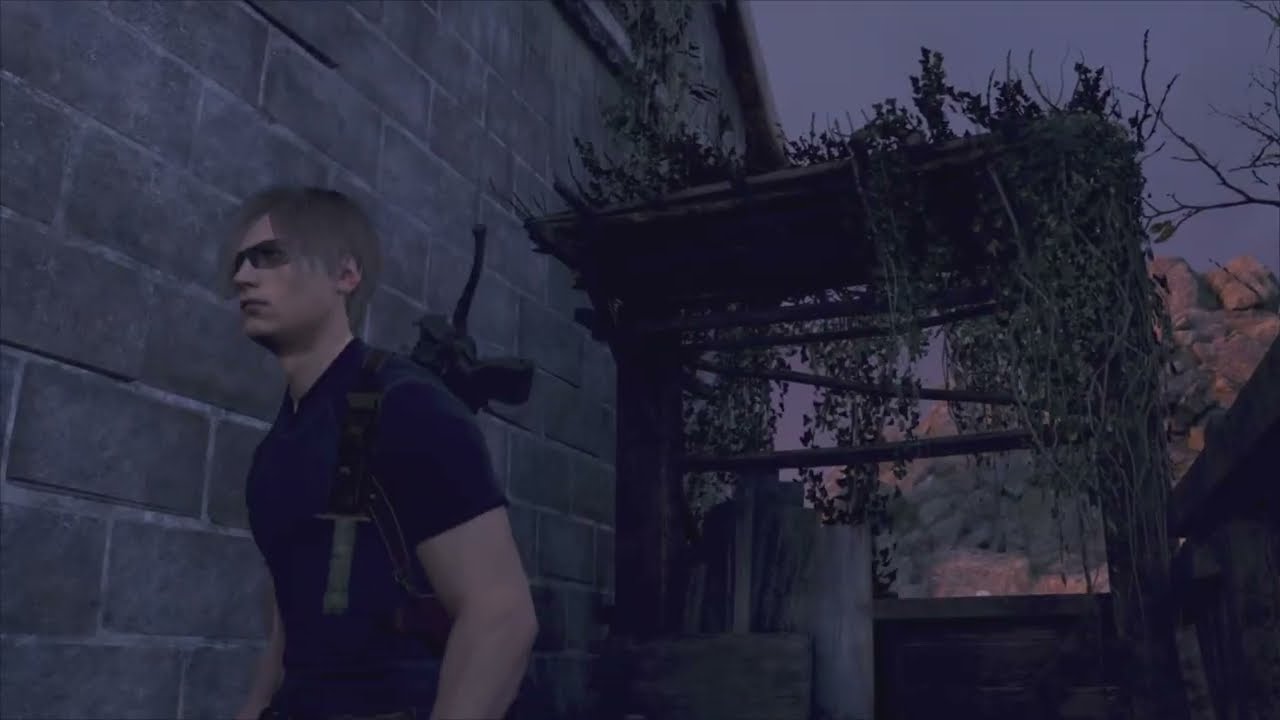In this detailed video game scene, a 3D-modeled character walks to the right, wearing a blue, short-sleeved t-shirt and dark sunglasses that obscure most of his face except his stern expression. His dark brown hair stands in contrast to a weapon, possibly a gun, strapped to his back. To his right, a concrete block wall defines the boundary of a nearby building. Directly behind him, a dilapidated wooden structure covered in lush, creeping plants and topped with a roof adds a touch of nature reclaiming the scene. Further back, a mountain bathed in sunlight rises in the distance, casting a warm light over the rugged landscape. The sky above is a tumultuous blend of grayish-blue hues, adding an atmospheric tension to the backdrop. The overall scene feels generated, with some odd textures and placements contributing to its surreal, otherworldly ambiance.